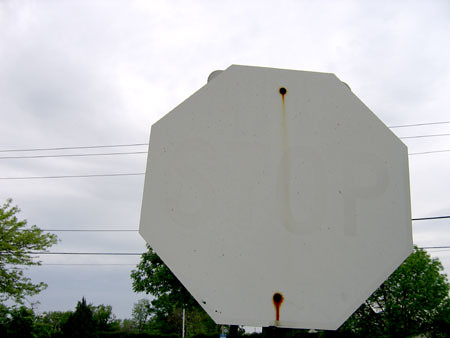This color snapshot photograph, taken outside on a somewhat cloudy but sunny day, prominently features an octagonal stop sign at the center of the image. The stop sign is entirely white, with the usual red background and STOP text completely eroded or faded from sun exposure, leaving only a barely visible shadow of the word "STOP." There are two screw holes at the top and bottom of the sign's face, each with rusty screws that have left brown rust streaks trailing down the surface. In the background, green trees and some telephone or electrical wires stretch horizontally across the center, contributing to the outdoor, suburban setting. The sky appears gray and overcast, adding to the overall faded and worn look of the image.